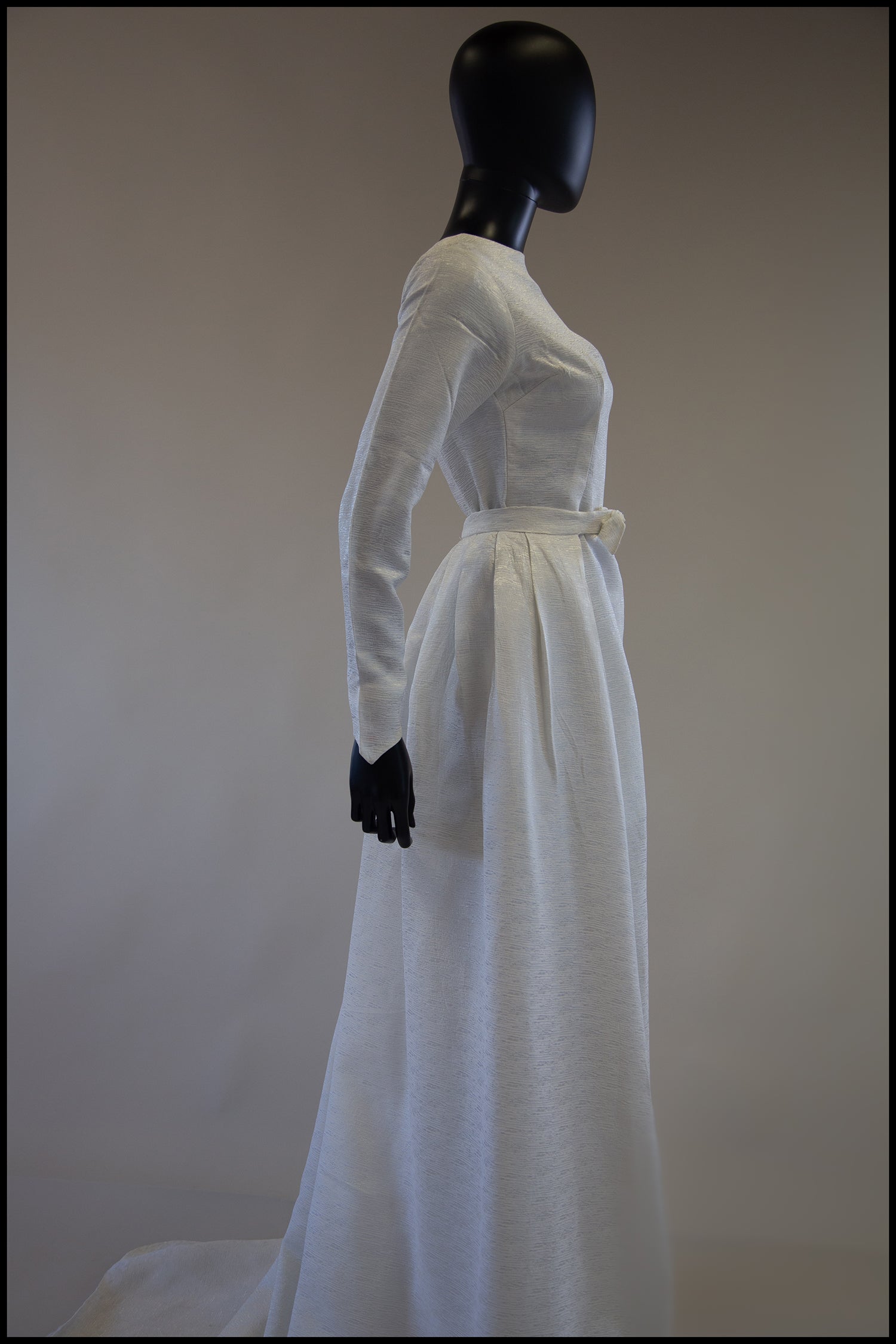The photograph features a matte black mannequin without facial features or hair, standing at an angle with its back slightly turned to the viewer. The mannequin is adorned in a long, flowing, floor-length white dress with a pleated skirt and long sleeves. A sash or ribbon cinches the waist of the dress, knotted elegantly at the front. The fabric of the dress appears thin, reminiscent of linen or a fine cotton. The scene is set against a simple, muted brown background, with the lighting creating delicate highlights on the front and sides of the dress, subtly emphasizing the shadows of the pleats despite an overall underexposure that makes the image somewhat dark. The gown evokes a vintage feel, potentially from an older era such as the 1930s or 1940s.